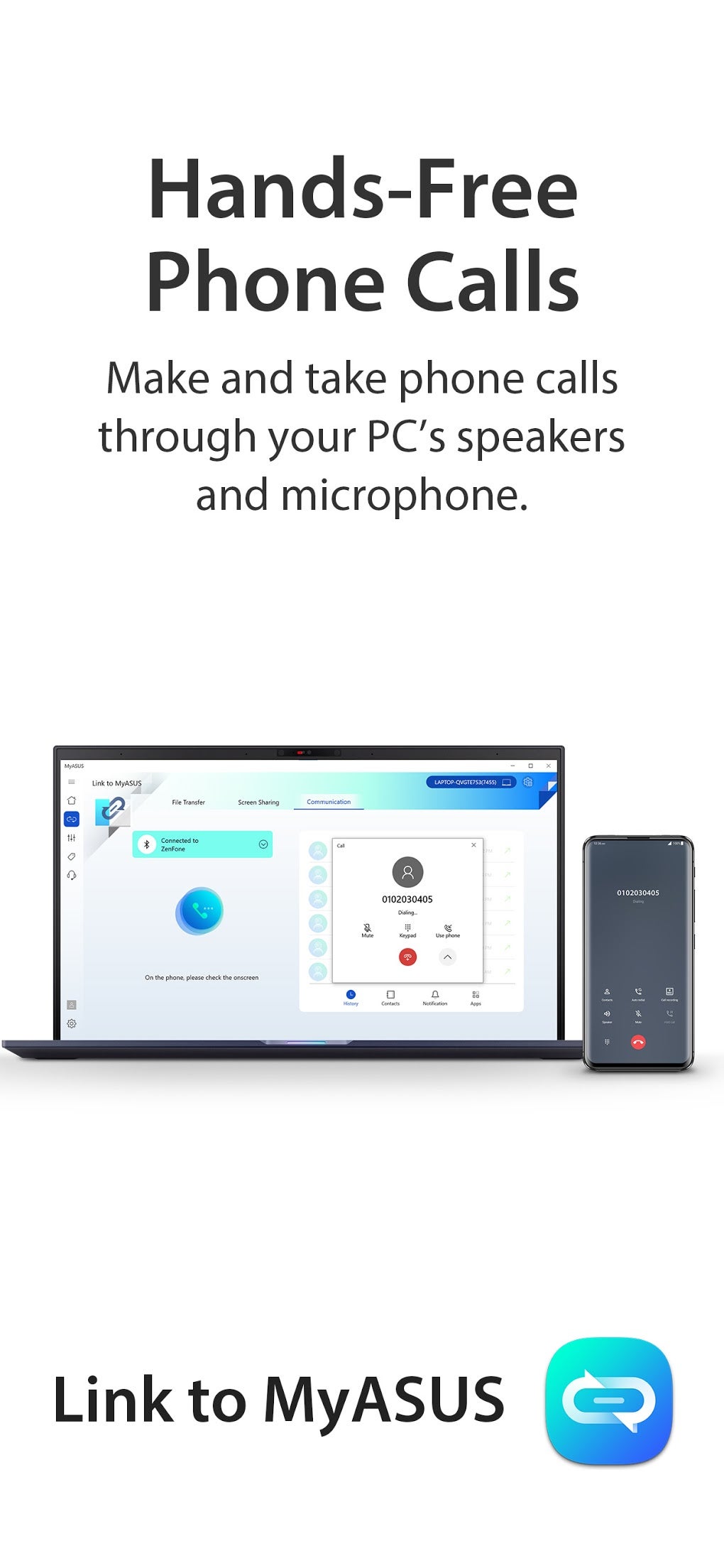### Hands-Free Communication Flyer Description

At the top center, bold black lettering prominently displays the phrase "Hands-Free," with both "H" and "F" capitalized. Below this, in slightly smaller but still bold black text, it says "Phone Calls." Even smaller, yet in the same font and color, it reads, "Make and take phone calls through your PC's speakers and microphone." Note that "PC's" is properly capitalized with an apostrophe 's.'

An image of a laptop is shown beneath this text. On the laptop screen, towards the top left-center, there is an aquamarine strip. At the bottom of this strip is a circular icon that transitions from dark blue at the bottom left to lighter blue at the top right. The icon has a shadow in medium navy blue, and small black writing appears at the bottom, seemingly forming a single phrase or sentence. Within the blue icon is a very light blue or aquamarine phone symbol.

To the right of the laptop image, there is a stretched-out cell phone graphic. The distortion makes it resemble a modem, but identifiable features such as the traditional red hangup button with a white phone pointing downwards clarify that it is indeed a phone.

At the bottom of the flyer, bold black text states "Link to MyASUS." Accompanying this text is a rounded symbol that fades from aquamarine at the top left to darker blue at the bottom right.